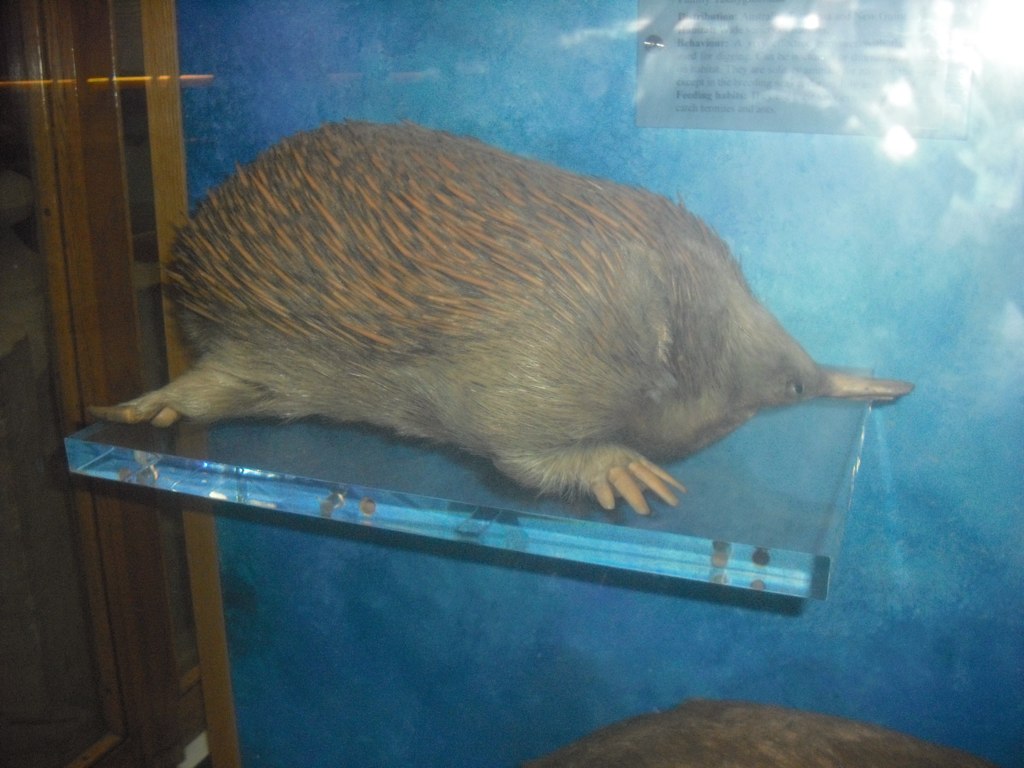This photograph, likely taken in a natural history museum, captures a taxidermied echidna displayed in a glass-fronted wooden case. The echidna, covered in brown quills with shades of orange highlights, lies flat on its stomach on a clear, thick glass shelf extending from a bright blue background. Its long snout, resembling a beak, points outward to the right, and its prominent claws are visible on both its front and back legs. A silver plaque providing information about the echidna is mounted on the blue wall above it, partially obscured by a camera flash reflected in the top right corner of the enclosure. Below the echidna, there appears to be another largely obscured taxidermied animal. The left side of the image features a wooden element, likely part of or adjacent to the display case.